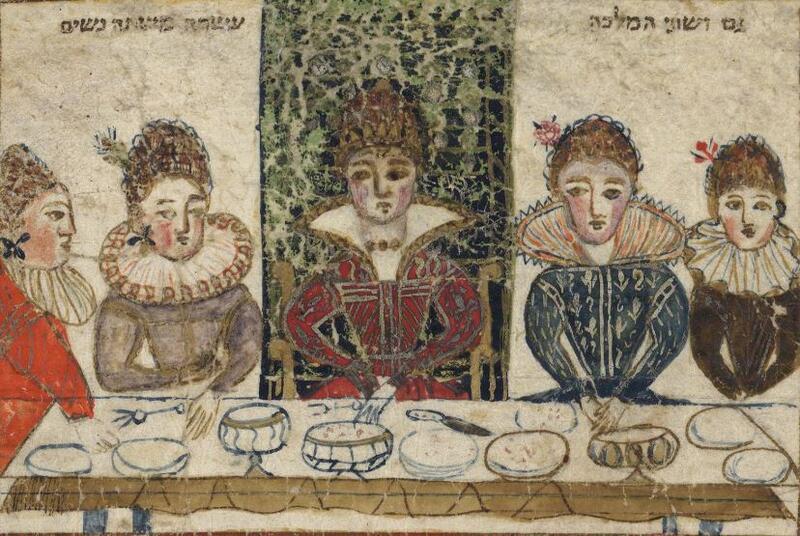Captured in an exquisite old-school painting or drawing on an antique scroll, this pre-Victorian era artwork depicts five regal women seated at a long dinner table adorned with plates, utensils, and likely servings of cheese and bread. Central to this composition is the Queen, distinguished by her elevated social status, as she sits on a special gold chair, wearing a striking red dress with an elaborate white collar fanning out from her neck, and a crown. She is the tallest among them and exudes authority. To her left, a woman in a long-sleeved purple dress sits, followed by another in orange attire. On the Queen's right, two women are dressed in blue and dark brown, respectively. All women have their hair elegantly styled in updos, decorated with roses and flowers, highlighting their nobility. Above the scene, ancient script resembling Judaic Hebrew complements the artwork’s antique aesthetic. The backdrop features a green and black tapestry, adding to the grandeur of the scene, though the women's serene expressions remain devoid of smiles.